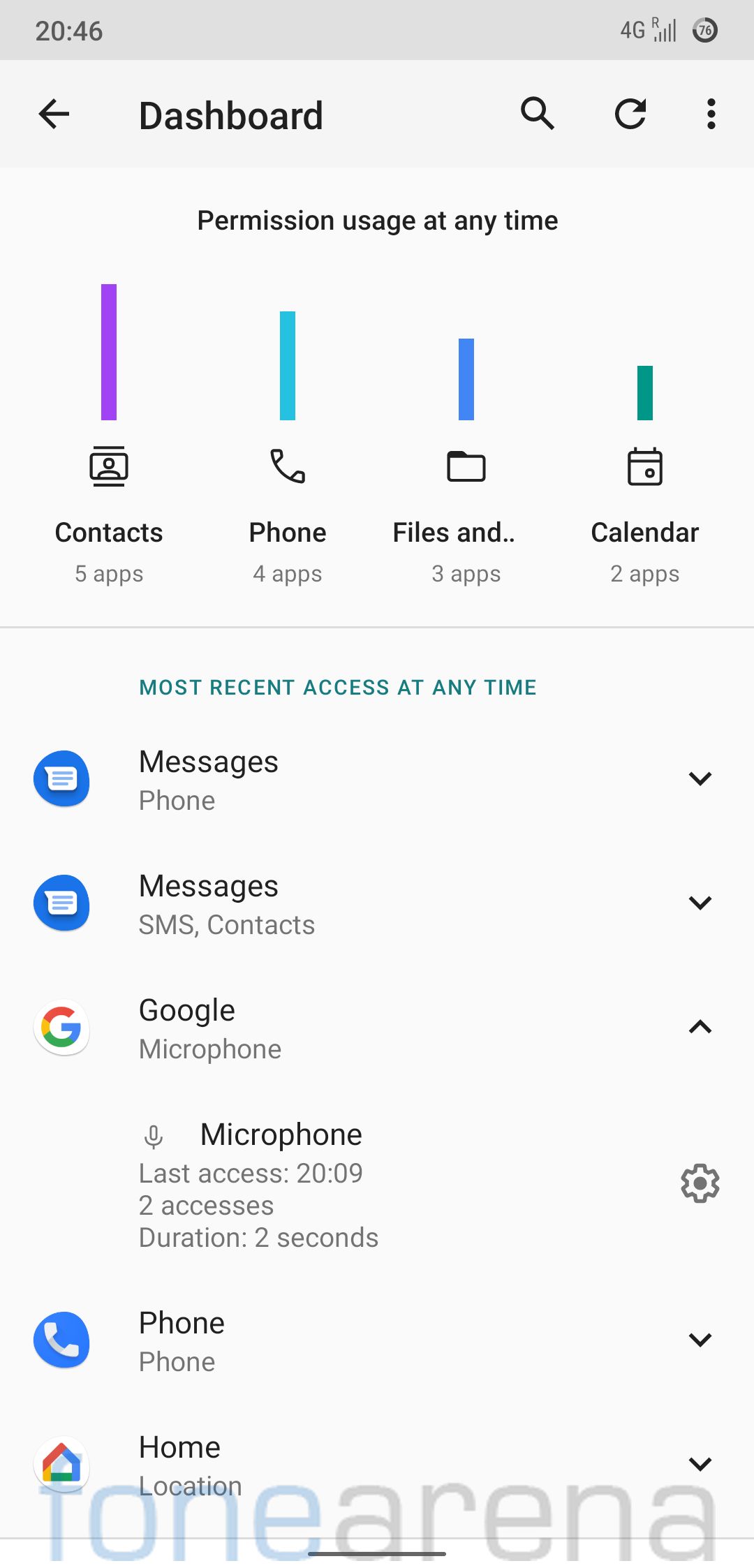This detailed screenshot image, taken on a smartphone, reveals various elements commonly found in a device's interface. In the top-left corner, the military time is displayed as 20:46 (8:46 PM), indicating a 24-hour time format. The status indicators show a strong 4G connection and full Wi-Fi signal strength.

The primary screen visible is a dashboard, marked by a black arrow pointing left towards the label "Dashboard." Adjacent to this label, there is a magnifying glass icon representing the search function, followed by a restart or refresh button, and the ellipsis (three-dot) menu icon.

Beneath the dashboard header, the section labeled "Permission usage at any time" showcases several categorized app groups with their respective usage information. The first icon represents contacts, denoted by a purple line, indicating the presence of five associated apps. Following this, the phone icon, highlighted by a blue line, shows usage details for four apps. The files icon, indicating three apps, and the calendar icon, representing two apps, are also displayed in this list.

Further down, under the section titled "Most recent access at any time," recent activities are shown with entries such as messages and phone, along with a drop-down menu for additional information.